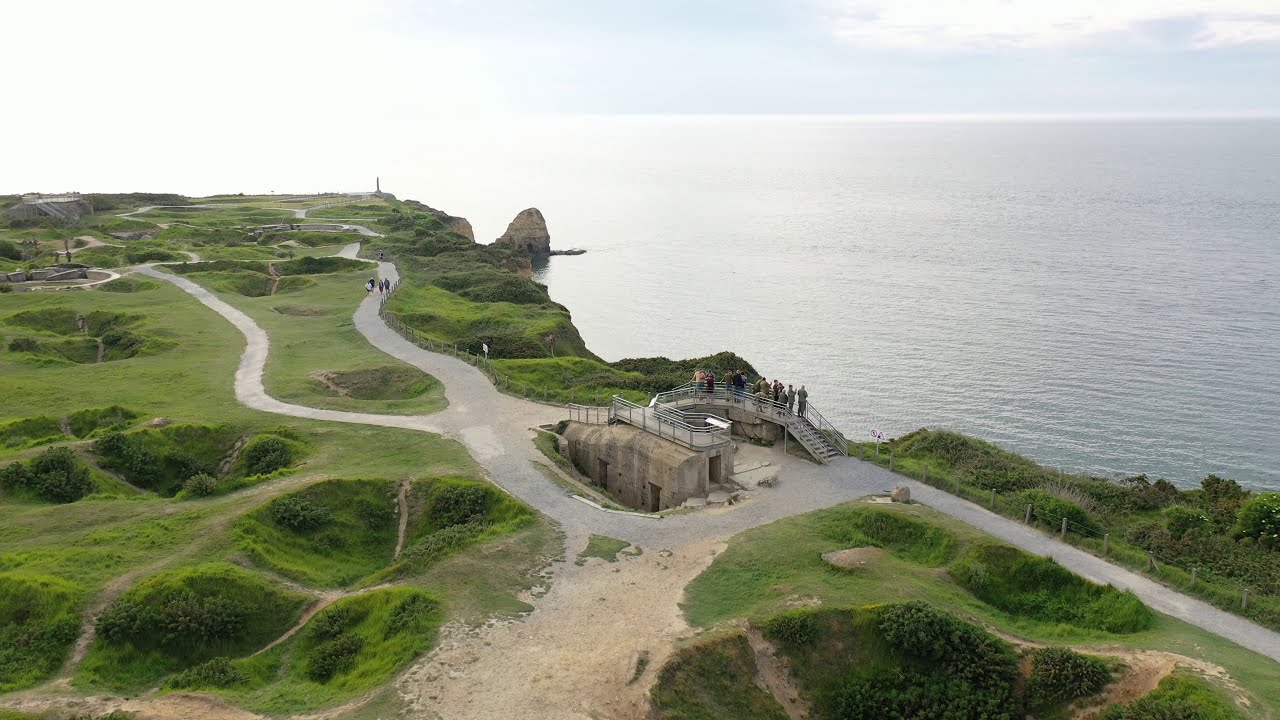This vibrant aerial photograph showcases a picturesque coastal landscape under bright blue skies adorned with fluffy white clouds. The scene is split between a lush, bumpy green terrain in the foreground and the expansive ocean that stretches to the horizon, where the sky meets the water in a beautiful gradient of blues and grays.

In the center of this landscape, a notable feature stands out: a circular paved turnaround area bordered by multiple walking paths. Three distinct, paved trails sprout from this central point, leading visitors through the verdant landscape. At the heart of the turnaround, there is a partially below-ground structure made of gray stucco, providing a base for an elevated walkway that crosses over the road, offering a spectacular vantage point overlooking the ocean.

This overlook area, complete with a bridge-like structure and fencing, allows people to take in the breathtaking coastal views and capture photographs. The scene is animated with individuals scattered along the paths, walking and enjoying the lookout point. Surrounding the central turnaround and paths, a network of paved roadways winds through the green expanse, connecting various parts of the landscape and leading back toward the landmass, ensuring smooth passage for exploration and return.

The photograph, taken from a drone's perspective, captures the essence of this serene roadside coastal overlook, emphasizing its harmonious blend of natural beauty and human-made paths and structures.